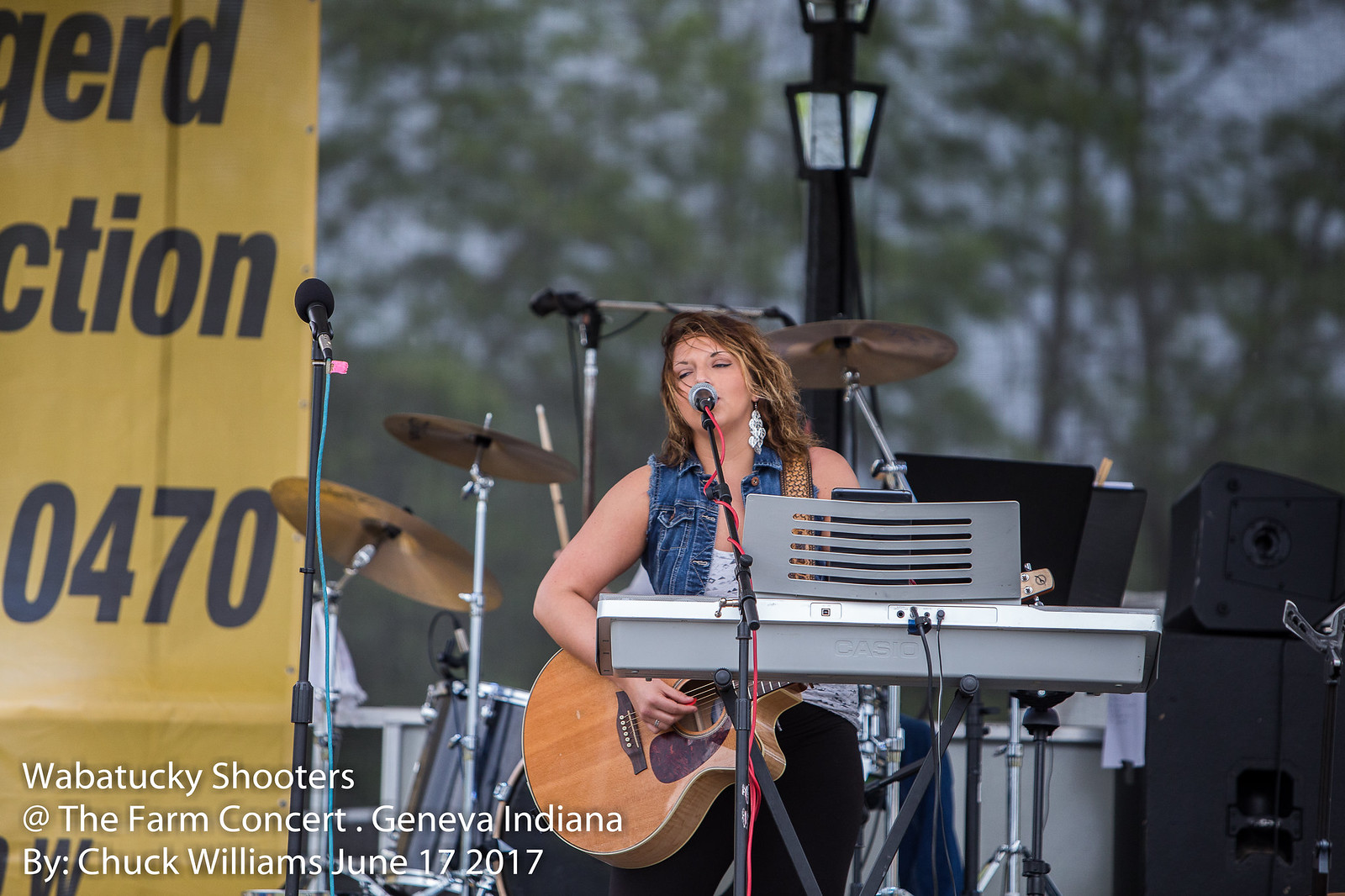A soulful image captures a beautiful woman on an outdoor stage, fully immersed in her musical performance. She’s strumming a light brown acoustic guitar, which is strapped around her with a wide, comfortable-looking strap. Dressed in a sleeveless, unbuttoned denim jacket over a light blue top and black slacks, she sits behind a gray Casio keyboard supported by a black stand. Her long brown hair flows freely, and she dons dangling white earrings, partially closed eyes suggesting she’s singing deeply into her microphone.

In the background, a drum set and a variety of percussion instruments, including cymbals and additional mics, surround her, hinting at a fuller ensemble. To her left stands a black light pole with a lamp, and beyond that, lush trees create a serene backdrop. On the right, a stack of black speakers stands ready to amplify her music.

A big yellow banner to her left reads partially, "G-E-R-D-C-T-I-O-N," possibly indicating a sponsor or event message. The scene is further detailed with white text in the lower-left corner which reads, "Wabatake Shooters at Farm Concert, Geneva, Indiana by Chuck Williams, June 17, 2017." Overall, it's an evocative snapshot of a captivating live performance on a summer day.